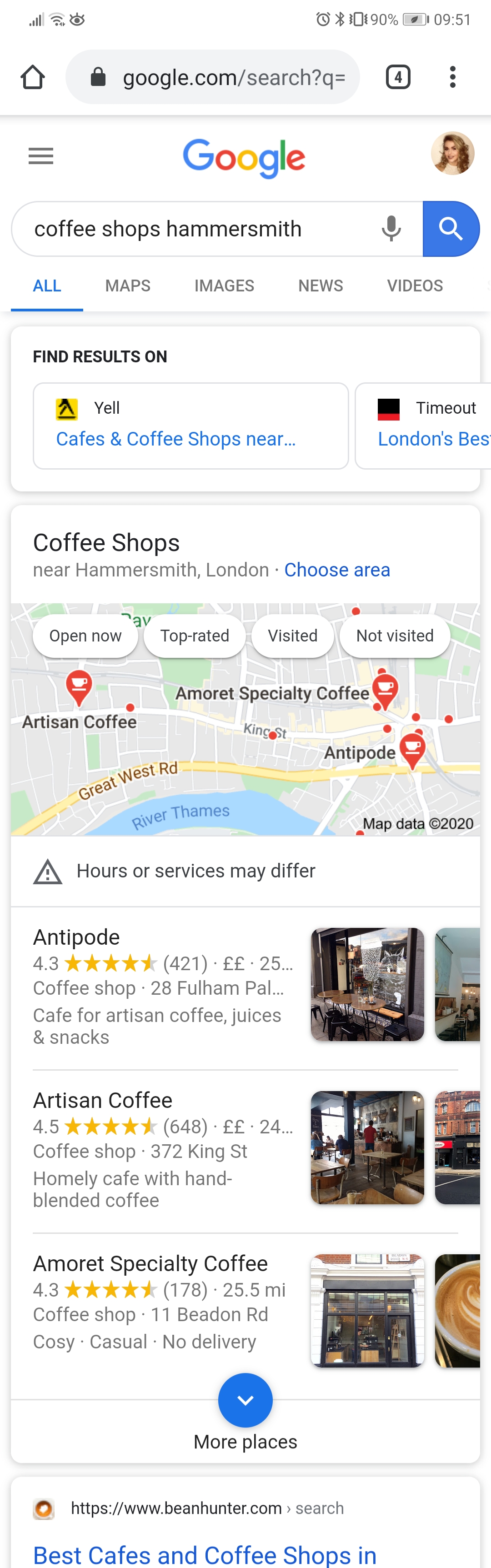A screenshot displays the results of a Google search for "coffee shops Hammersmith" on a mobile device. The search bar at the top is highlighted in blue, with a small microphone icon indicating voice search capability. Below the search bar, there are tabs labeled "All," "Maps," "Images," "News," and "Video."

The search result page features multiple sections. The first section showcases links to related resources such as Yellow Pages and specific categories like "Cafes and Coffee Shops." This is followed by highlighted search results stating, "Coffee shops near Hammersmith, London," and options to refine the search by "Choose area," "Open now," "Top rated," "Visited," and "Not visited."

A map displays numerous pin markers, each adorned with a coffee cup icon, indicating the physical locations of coffee shops. There is a note mentioning, "Hours of service may differ," alongside a list of three specific coffee shops: Antipode, Artesian Coffee, and Amaro Specialty Coffee. Below this list, there is a blue button labeled "More" to load additional search results.

The bottom part of the screenshot includes six small images showcasing different aspects of a coffee shop and a latte. The map data is dated from 2020. At the top right corner, a partial view of a person’s profile photo is visible, along with a battery status indicating 90% charge remaining.